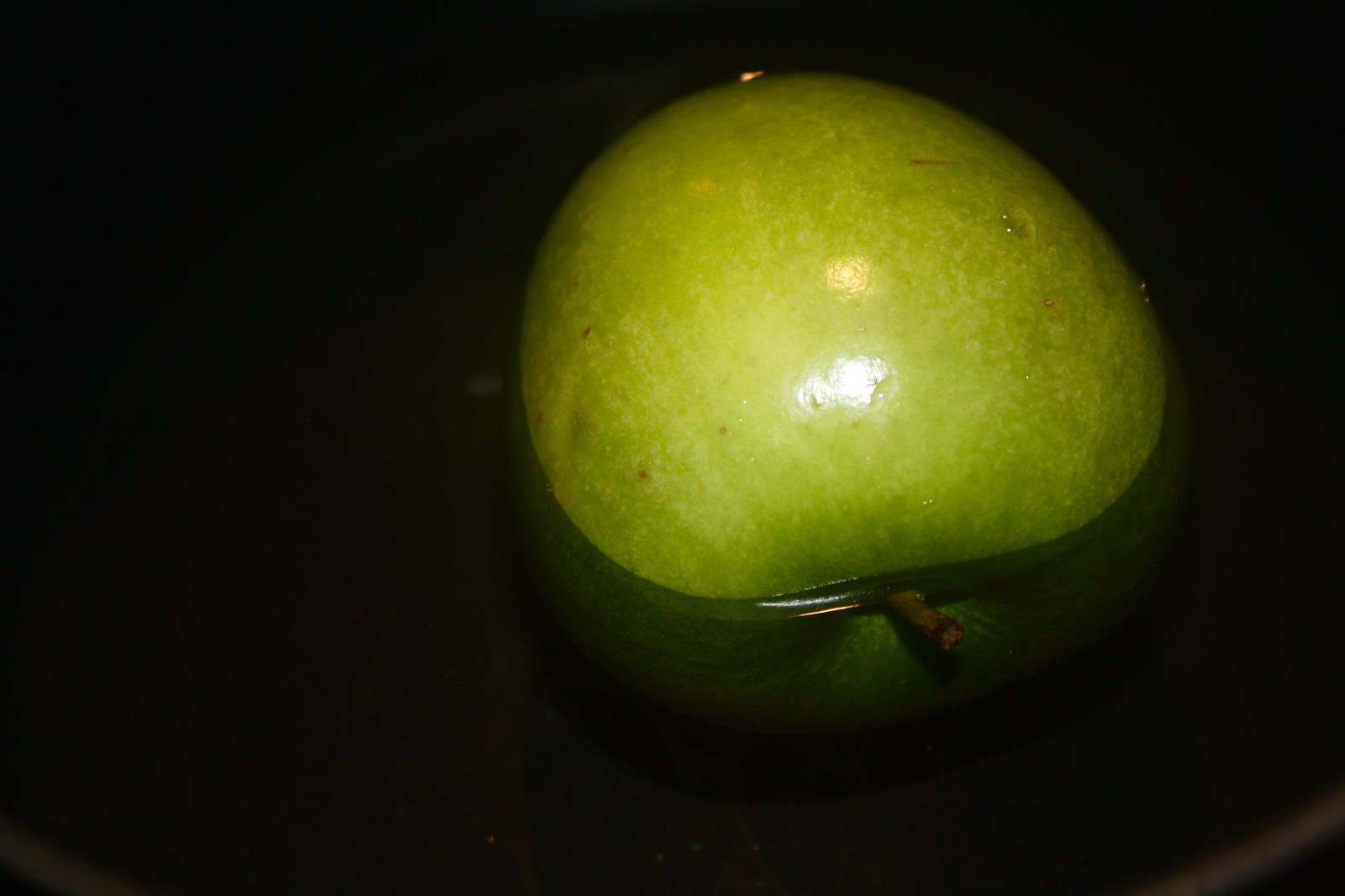The photograph captures a minimalist composition featuring a sleek black bowl, occupying the majority of the frame. Accenting the base of the bowl are two subtle white-gray lines located on the bottom left and right sides. The bowl is filled with clear water, providing a reflective surface that enhances the visual appeal of the scene.

Centrally placed within the bowl floats a vibrant green apple, speckled with tiny white dots and accented by subtle black lines and brownish spots. The top of the apple features two distinct sun glares: a larger, prominent one and a smaller, more delicate one, adding a touch of sparkle to its surface. The apple is partially submerged, with the water level rising slightly past its midpoint. At the top of the apple, a small brown stem is visible, partially submerged beneath the clear water, adding a naturalistic detail to the composition.